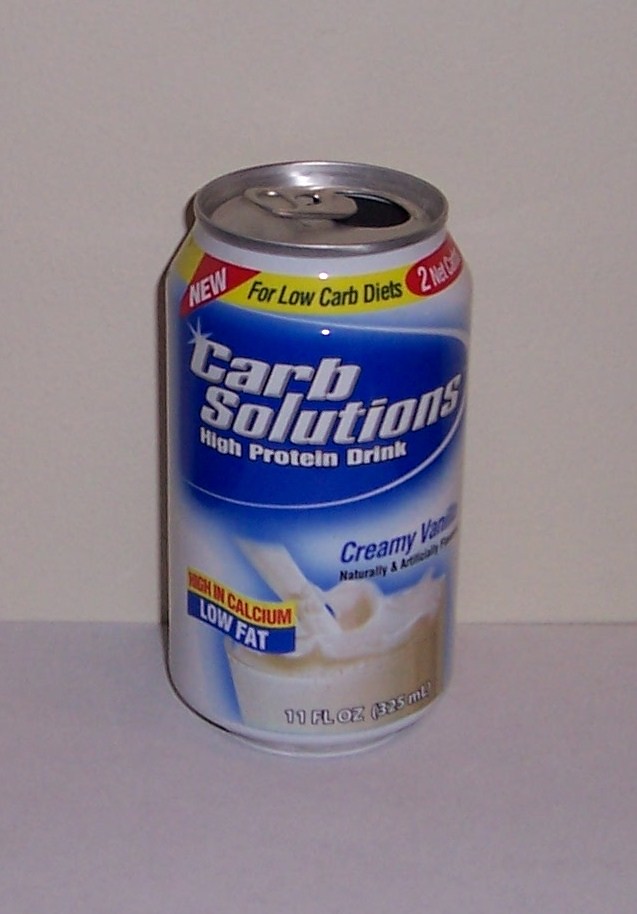The rectangular photo showcases a can placed on a gray table or counter. The can, with its flip-top lid open, prominently features a branding design in red, white, and blue against a blue background. "Carb Solutions" is written boldly in white print, with "High Protein Drink" in smaller, white letters below it. An image of the top of a vanilla shake, complete with a white straw, decorates the front of the can. Next to this image, blue print reads "Creamy Vanilla Naturally and Artificially Flavored." Additionally, across the vanilla shake image, red print says "High in Calcium," and white print states "Low Fat." Above the brand name, the top of the can indicates "For Low Carb Diets" and highlights "New 2 Net Carbs."